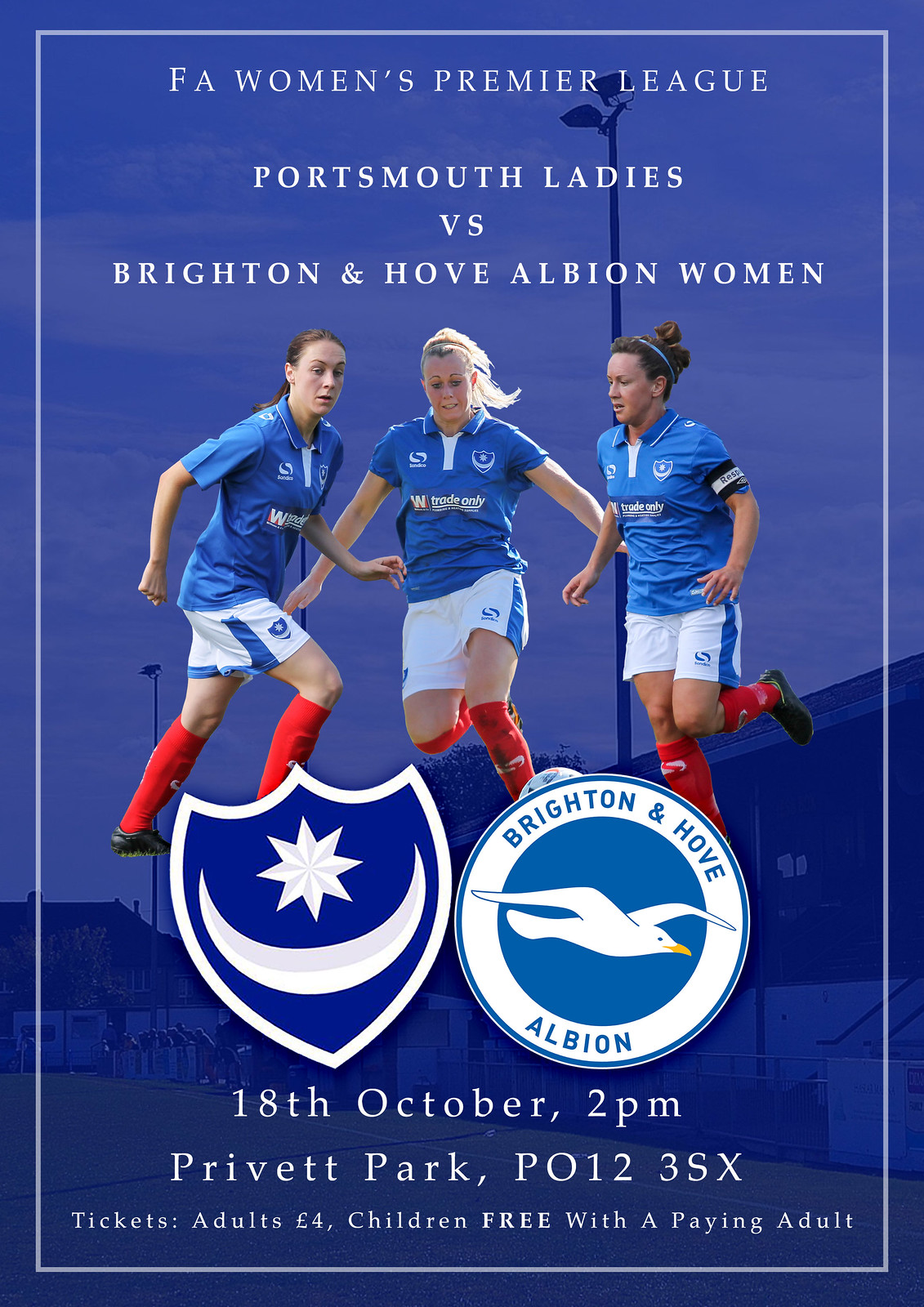The promotional poster for the F.A. Women's Premier League match between Portsmouth Ladies and Brighton & Hove Albion Women features a striking blue-filtered background image of a soccer field with an empty stadium. The entire poster is bordered by a light gray line and contains several prominent elements. At the top, in bold white text, it reads "F.A. Women's Premier League Portsmouth Ladies versus Brighton and Hove Albion Women." 

Below the text are photographs of three soccer players in action, each wearing a blue jersey, white shorts with a blue stripe, and red shin guards. Beneath the images of the players are two contrasting logos: on the left, a shield featuring a white star and crescent moon with a blue background, and on the right, a circular logo depicting a flying seagull against a blue backdrop with the text "Brighton & Hove Albion." 

Additional event details are provided in white text towards the bottom of the poster: "18th October, 2pm, Privet Park, P.O. 12, 3SX. Tickets adults £4, children free with a paying adult." This comprehensive and visually appealing flyer effectively promotes the upcoming soccer game, highlighting key information and imagery.